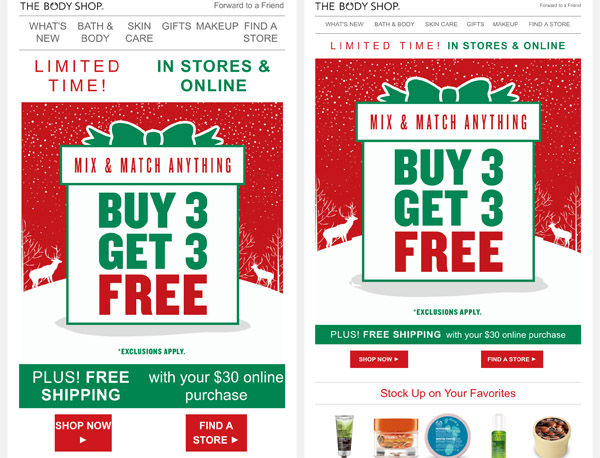This image showcases two advertisements from The Body Shop, both prominently displaying the brand's name in black letters at the upper left-hand corner. Beside the brand name, there's a hyperlink allowing users to forward the ad to a friend. Below this, a navigation bar features five hyperlinks: "What's New," "Bath and Body," "Skin Care," "Gifts," and "Makeup," along with an additional button to locate a nearby store.

The primary ad promotes a "Buy 3, Get 3 Free" Christmas offer, adorned with festive red and green colors and reindeer illustrations. This main ad does not include product images. The secondary ad, smaller in size to accommodate five product thumbnails, encourages customers to "Stock Up on Your Favorites." The displayed products include a cream, a lotion, a facial scrub, a body mist, and bath salts, respectively.

Overall, the ads combine festive elements with practical product highlights to attract holiday shoppers.